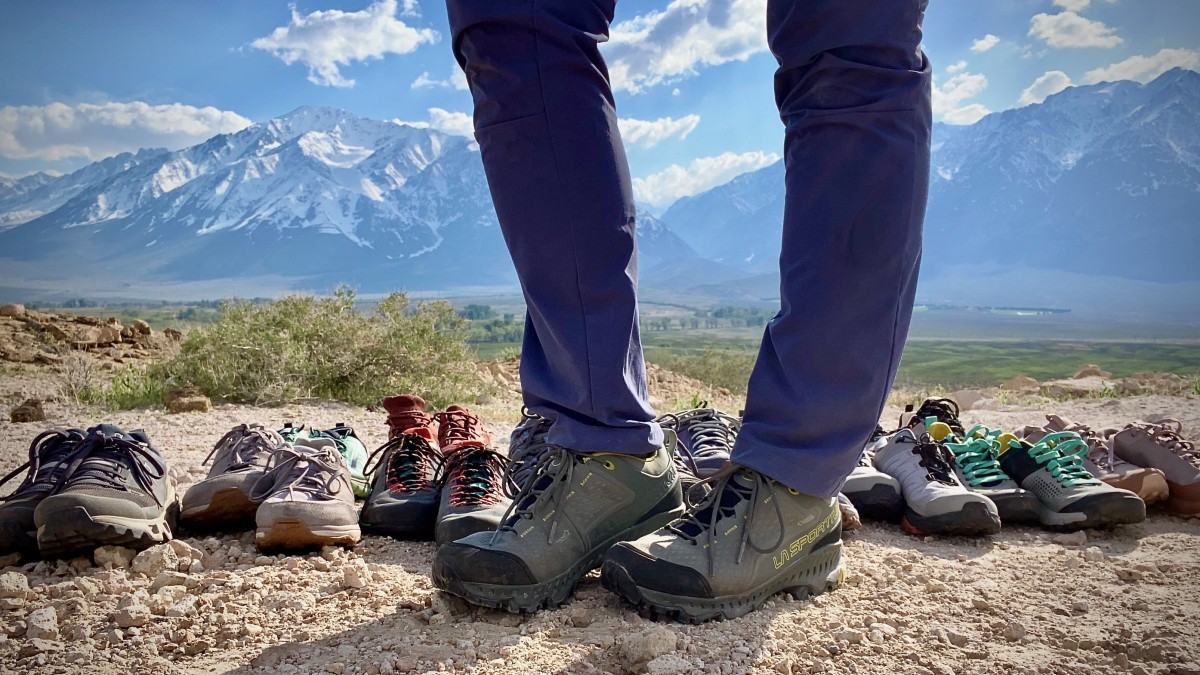This captivating nature shot features a close-up of a man's legs and feet, clad in blue pants and gray hiking shoes accented with yellow trim and black toes, standing on a gravel surface. Behind him, a diverse line of hiking shoes of various colors and styles, including shades of gray, tan, orange, beige, and black with different detailing such as red accents and green laces, are neatly arranged. The scene is set against a stunning backdrop of snow-capped mountain ranges, illuminated by the sun, and a vibrant blue sky dotted with fluffy clouds. The background also includes a grassy dune leading into a lush valley with distant trees, adding depth and a sense of adventure to the overall composition.